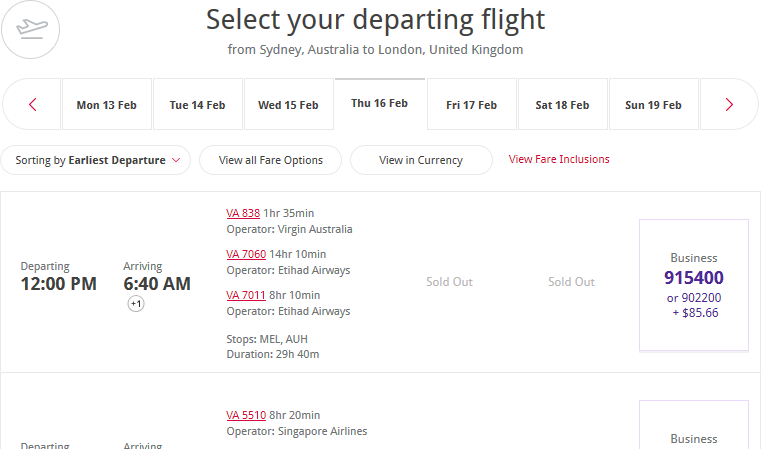The image displays a flight selection screen for a departing flight from Sydney, Australia to London, United Kingdom. At the top, a header prompts users to "Select Your Departing Flight from Sydney, Australia to London, United Kingdom." Beneath this, a date range from Monday, 13th February to Sunday, 19th February is shown, with clickable options for each day. Below this date range, there is a sorting option labeled "Sort by Earliest Departure," a "View All Fare Options" button, and another button for choosing currency labeled "View in Currency."

A red hyperlink titled "View Fare Inclusions" is also present. Following this, two white rectangular boxes display specific flight details. The first box indicates a flight departing at 12:00 PM and arriving at 6:40 AM. It lists flight numbers VA 838 (operated by Virgin Australia, duration 1 hour 35 minutes) and VA 7060 (operated by Etihad Airways, duration 14 hours 10 minutes). The second box mentions flight VA 7011 with a flight duration of 8 hours 10 minutes.